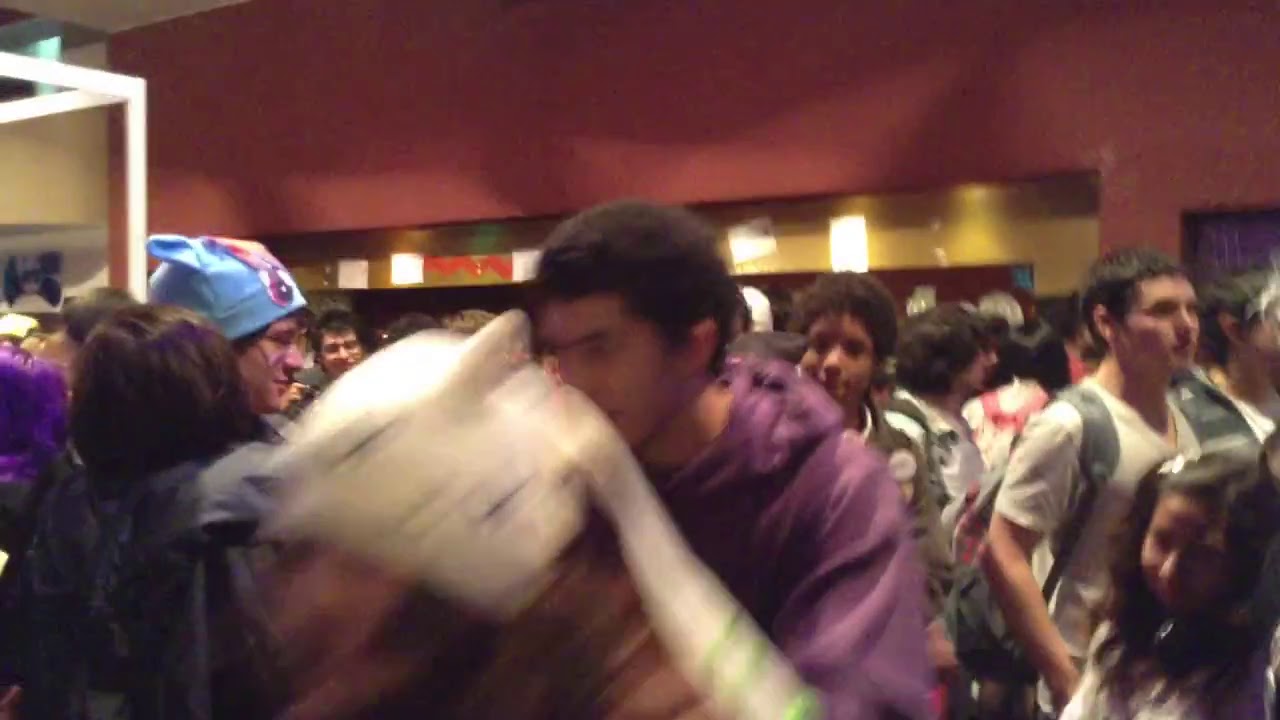The image depicts a bustling indoor scene at what seems to be a school or convention, filled with young individuals, both male and female, carrying backpacks. The majority appear to be teenagers, with a diverse mix of black and white individuals. The setting is highly crowded, probably with around 40 people, all navigating through what looks like a hallway or a reception area.

The background features a maroon-colored upper wall transitioning into a gold or yellow-colored section beneath it, where pages or notes are taped. The lower part of the scene resembles a reception area or stand, embellished with gold trim and pillars, suggesting a more formal or organized venue.

A notable element in the foreground is a person with a blurred face wearing a distinctive white hat with long ears, resembling bunny ears or an anime-inspired accessory. Standing behind them is an individual in a purple hoodie with short black hair. The entire image is characterized by low quality, digital noise, and compression artifacts, making many details soft and unclear.